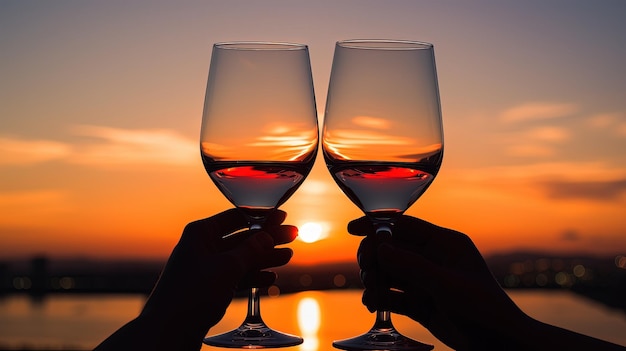Against a stunning sunset backdrop, this photograph captures two people toasting with large wine glasses, partially filled with red wine, creating a captivating silhouette effect. The hands holding the glasses—one appearing more feminine, the other more masculine—are mostly in shadow, with a slight hint of subsurface scattering visible on a finger of the left hand. The wine glasses, clinking together just slightly off-center above the glowing horizon, magnificently distort the scene within them due to refraction, flipping the captured image upside down. The sunset paints the sky in a gradient of warm oranges transitioning into dusky blues, reflecting beautifully in the calm body of water below. Twinkling lights from what appears to be a small town or city flicker in the distance, adding a sense of enchantment to the serene evening setting. The overall composition balances the dynamic interplay of natural light and delicate reflections, creating a picturesque and celebratory moment.